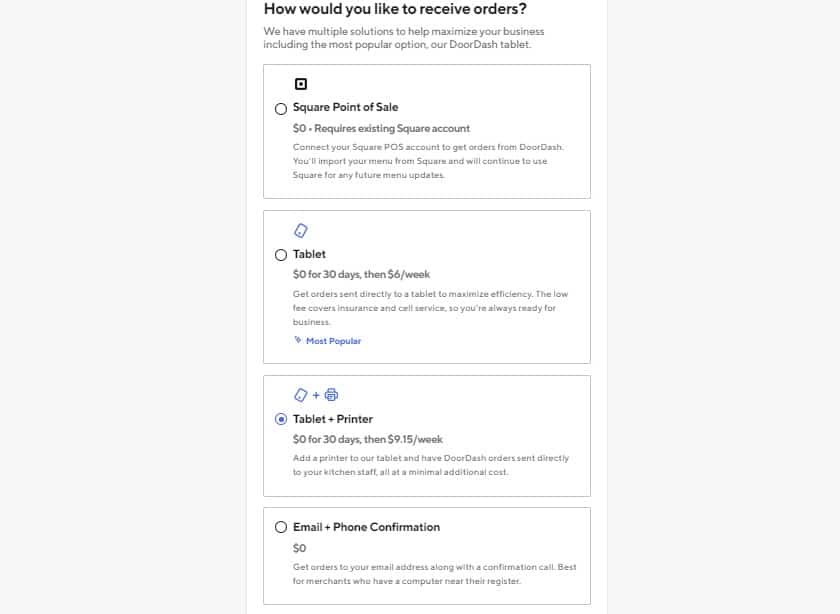The screenshot features a section of a website dedicated to order receiving options. At the top, a bold black header asks, "How would you like to receive orders?" followed by a subheading in gray text stating, "We have multiple solutions to help maximize your business including the most popular option, our DoorDash tablet."

Beneath this, there are four selectable options displayed as boxes with accompanying bubbles for choosing preferences. The third option is checked, indicating "Tablet + Printer." 

1. **Square Point of Sale** - Listed at the top, this option is marked as $0 and states that it requires an existing Squares account. There is additional, small, unreadable text.
   
2. **Tablet** - This unchecked option is highlighted in black text, offering a promotional price of $0 for the first 30 days, followed by a charge of $6 per week.

3. **Tablet + Printer** - The selected option shows in black at the bottom: $0 for 30 days, then $9.15 per week. Like the others, it contains some small, unreadable text in gray below the cost details.

4. **Email and Phone Confirmation** - Located beneath the selected "Tablet + Printer" option, this is also in black text and marked as $0. Two sentences of small, unreadable text are displayed beneath it in gray.

The left and right sections of the screenshot are plain and wide, devoid of any content, emphasizing the central focus of the webpage.